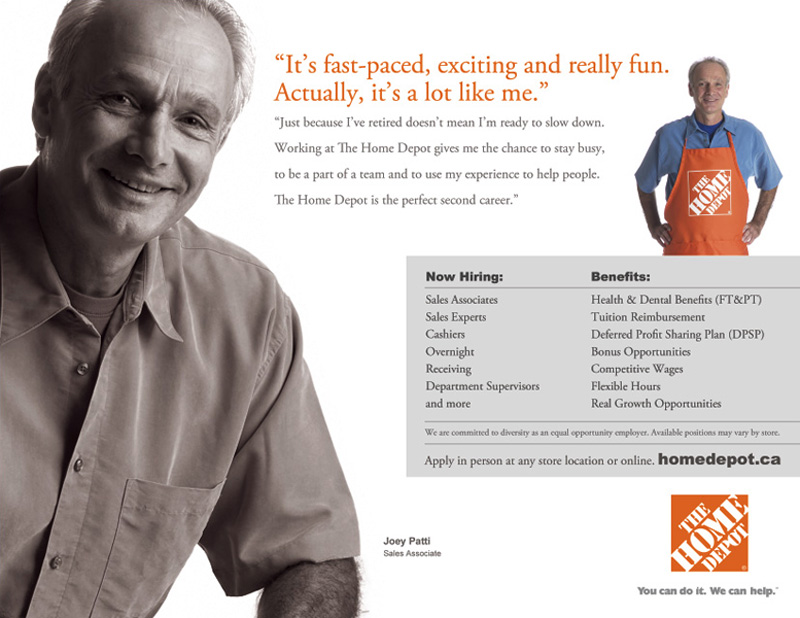The image is a digital advertisement for hiring by The Home Depot, featuring Joey Patti, a retired but actively working sales associate. The background is white, and the main focus on the left side is a large black-and-white upper-body photo of Joey Patti, an older Caucasian man with a receding hairline and gray hair, smiling warmly at the camera in a collared shirt. To the right of his black-and-white image is an orange-text quote from Joey that reads, "It’s fast-paced, exciting, and really fun. Actually, it's a lot like me. Just because I've retired doesn't mean I'm ready to slow down. Working at The Home Depot gives me the chance to stay busy, to be part of a team, and to use my experience to help people. The Home Depot is the perfect second career." Beneath this quote, in smaller gray text, additional details about the job's benefits and positions are provided.

Further to the right, there is a smaller color image of Joey wearing an orange Home Depot apron. Below this color photo is a prominent gray box that outlines the different hiring locations, available positions, and associated benefits. In the bottom right corner of the image, the iconic Home Depot logo is displayed in its recognizable orange and white colors, with the slogan "You can do it, we can help" written beneath in gray font.